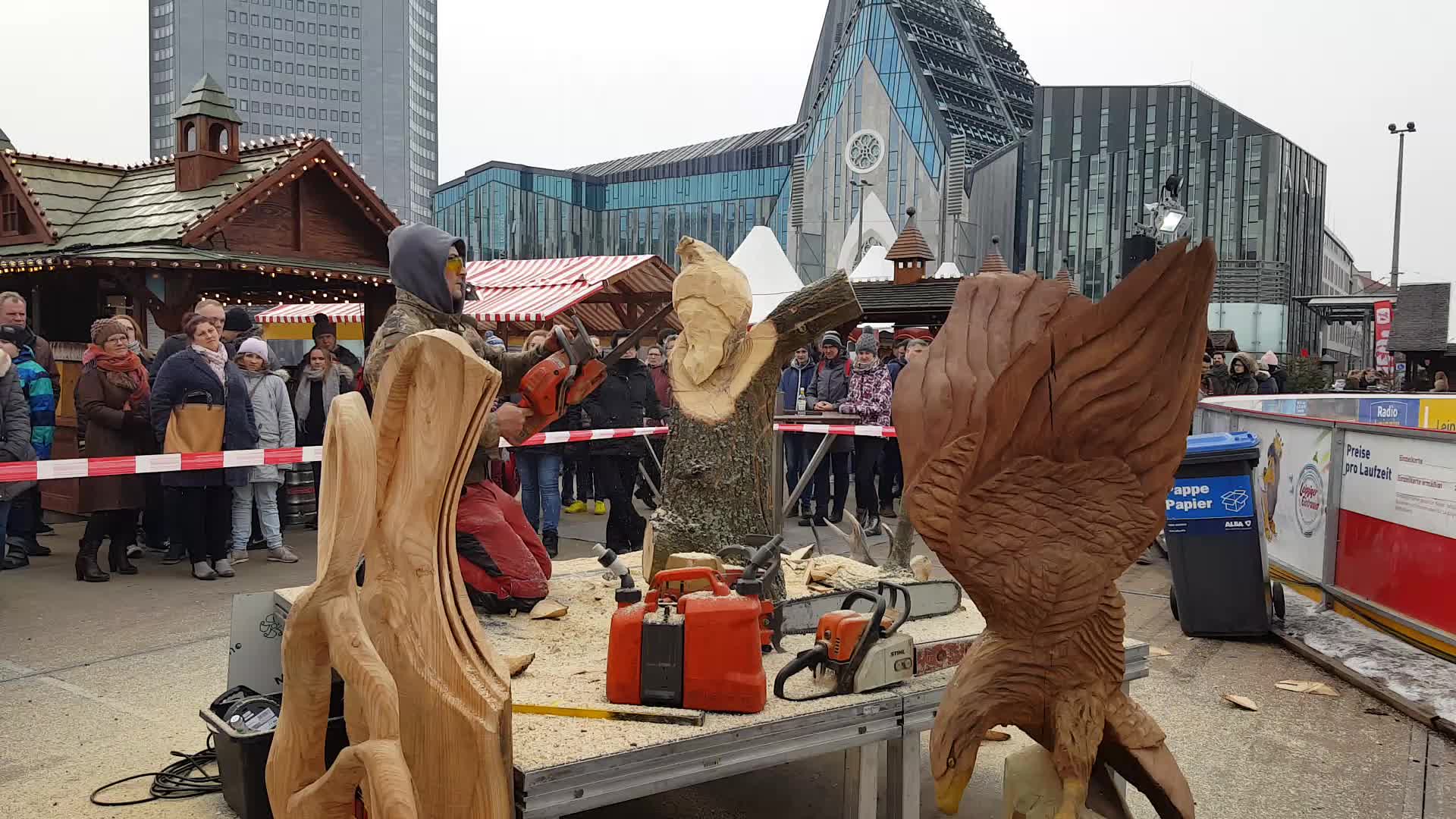The image depicts a bustling scene at the center courtyard of a carnival or festival, cordoned off by red and white tape. The main focus is a rustic wooden table at the center, adorned with various tools including a small red and black gas can and several red, white, and silver chainsaws. Engaged in a burst of creative activity, a man is in the process of chainsaw carving a large circular log positioned on the table. Intricate wood carvings, including an eagle-like bird diving into water and another ambiguous tan piece, are showcased to the bottom right and left of the table. Nearby, an imposing black bear carving with an outraised arm and a fantastical figure with wings and multiple legs are also visible. Separating the workspace from onlookers, a crowd is gathered around, intently watching the craft unfold. In the background, various wooden-topped huts and booths typical of a carnival add to the festive atmosphere, while larger, modern buildings, including a tall silver-colored structure and a sleek glass-and-blue architectural marvel, loom overhead under a light gray sky, further framing this vibrant scene.